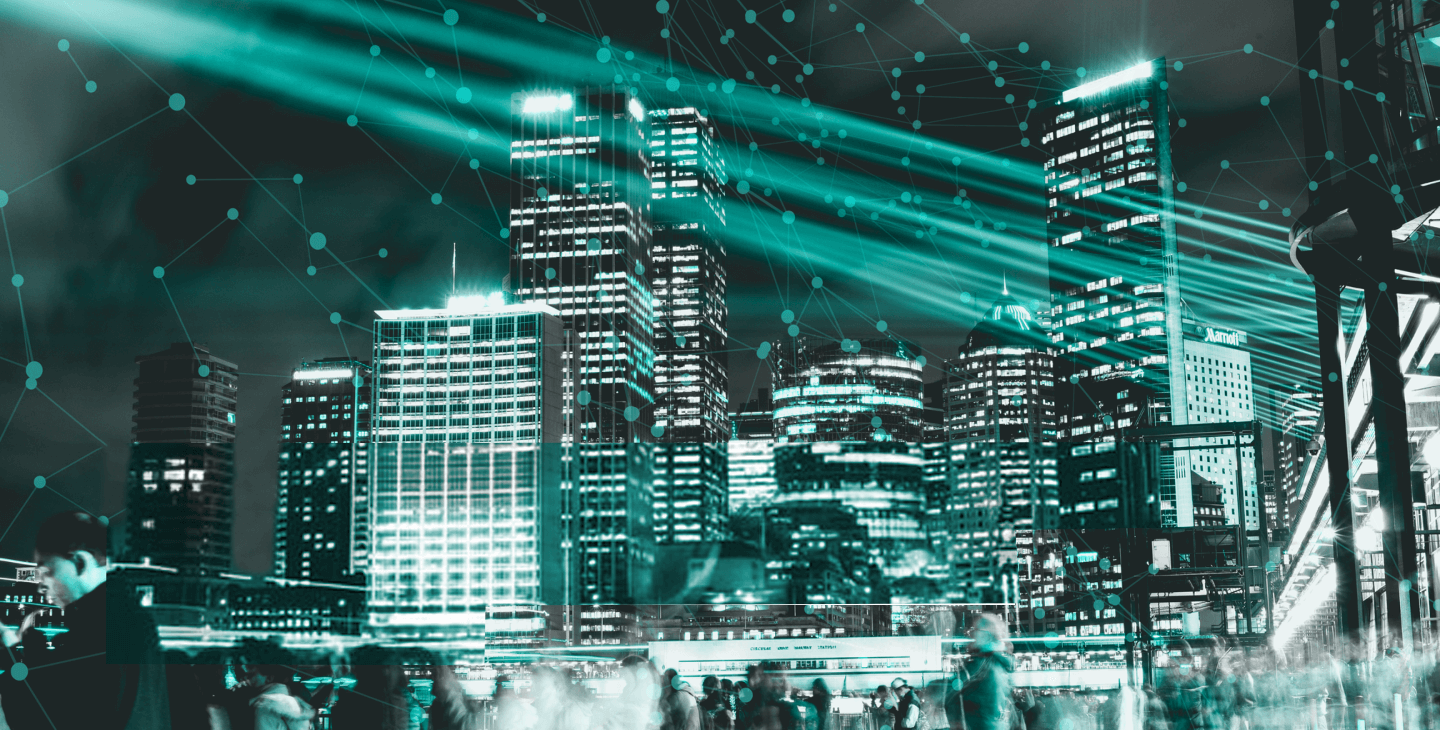This digitally manipulated, futuristic sci-fi cityscape radiates an ethereal glow against the night sky. Originally a black and white photograph, it has been altered with vibrant teal hues that highlight the illuminated windows of towering skyscrapers. These buildings dominate the skyline, juxtaposed against a cloudy night sky with a subtle gradient of dark green tones.

In the foreground, a bustling street scene reveals people clad in coats, some appearing blurred due to a long exposure. This gives the scene a dynamic energy, capturing the constant motion of urban life. An array of interconnected, light blue constellation-like designs overlay the scene, weaving a web-like pattern that connects the various elements of the image. Horizontally oriented beams of teal light—reminiscent of laser beams—cut across the composition, emerging from buildings on the right and stretching toward the top left, adding depth and a sense of futuristic technology. Despite its high realism, the digital manipulation imbues the image with a distinctly otherworldly atmosphere. Unreadable text in the background hints at hidden stories within the city, enhancing the enigmatic allure of this nocturnal metropolis.